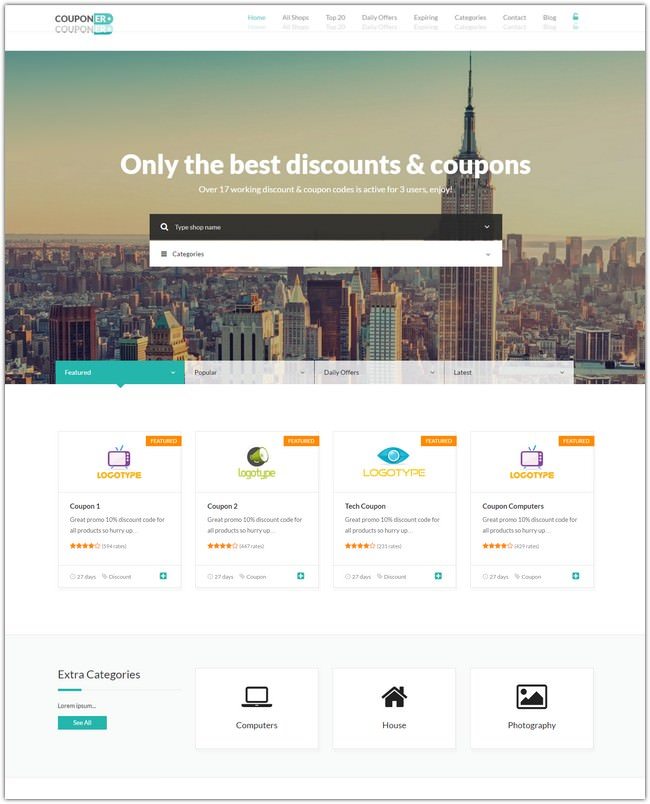In this image, we see a well-designed webpage belonging to a website named "Couponer." The top navigation bar features several drop-down menus labeled "Home," "All Shops," "Top 20," "Daily Offers," "Expiring," "Categories," "Contacts," and "Blog." The focal point of the page includes a vibrant cityscape, showcasing high-rise buildings in the background, which gives the site a dynamic and urban feel.

Central to the page is a prominently displayed search field labeled "Type shop name," accompanied by a drop-down menu titled "Categories." Above this, a banner headline boasts, "Only the Best Discounts and Coupons." An additional message highlights that over 17 working discounts and coupon codes are currently active, available for three users to enjoy.

Below the search field, various categorized options such as "Coupon One," "Coupon Two," "Logo Type," "Coupon Three," and "Buy Logo Type" are organized and easily accessible. Additionally, categories listed include "Take Coupon," "Coupon Four," "Coupon Computers."

Towards the bottom of the page, extra categories such as "Computers," "House," and "Photography" are available for users to explore further.